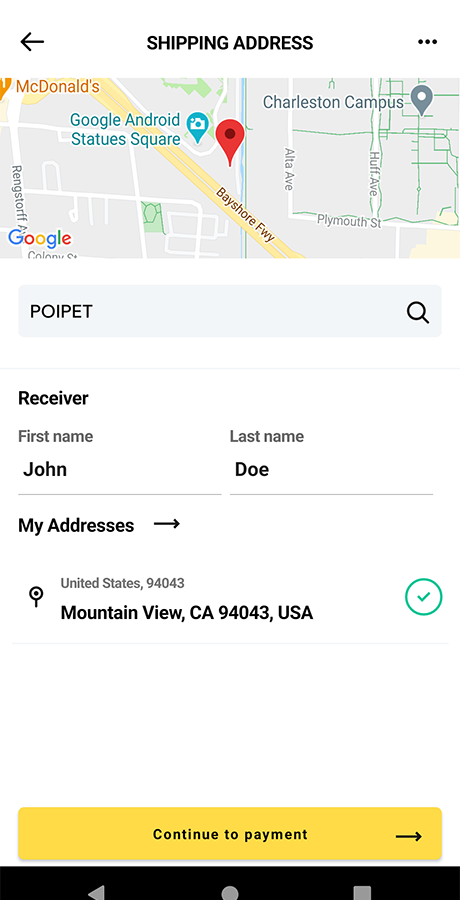Screenshot displaying a search for the POIPET location, highlighted on a map with a prominent red marker. The displayed address is situated in Mountain View, California, with the postal code 94043. It is located between the notable landmarks of the Google Android Statue Square and the Bayshore Freeway, specifically west of the Charleston campus.

The image includes details of a potential shipping address, associated with the receiver named John Joe. A green checkmark indicates the address's eligibility or confirmation. At the bottom of the screenshot, there is an option to "Continue to Payment," along with navigation bars providing "Get back home" and "Menu" buttons. The primary focus is on the precise positioning and validation of the Mountain View address for shipping purposes.